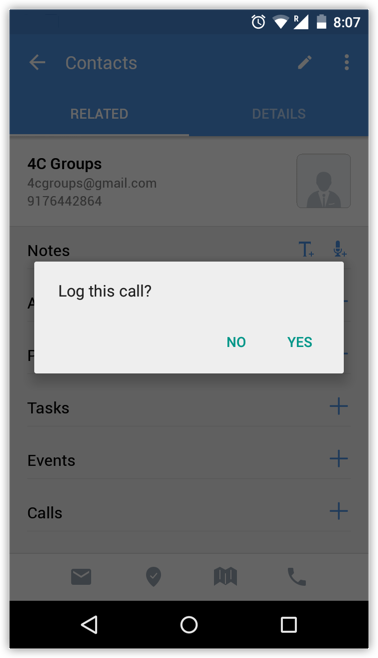A detailed screenshot of a smartphone's contacts panel. Most of the screen is dimmed because of a prominent pop-up window in the upper left corner that reads "Log this call" within a white rectangle. Directly below this, in the lower right corner, are teal green buttons labeled "No" and "Yes" for user response. 

At the top right of the screen, the time is displayed as 8:07, accompanied by status icons from right to left including a battery icon showing around 50% charge, full signal strength, Wi-Fi connectivity, and an alarm clock icon.

The contacts panel beneath the pop-up window displays information for a contact associated with the email address 4cgroups@gmail.com. There is a placeholder profile picture showing no image, and the phone number listed as 417-644-2864. Additional details such as notes are partially obscured by the pop-up window.

Further down, there are sections labeled "Tasks" with a blue plus button on the right, "Events," and "Calls." At the very bottom of the screen is a navigation menu, featuring icons for email (an envelope), location mapping (a map pin), and calling (a telephone receiver). The standard three-button navigation bar with a black background completes the interface at the bottom.